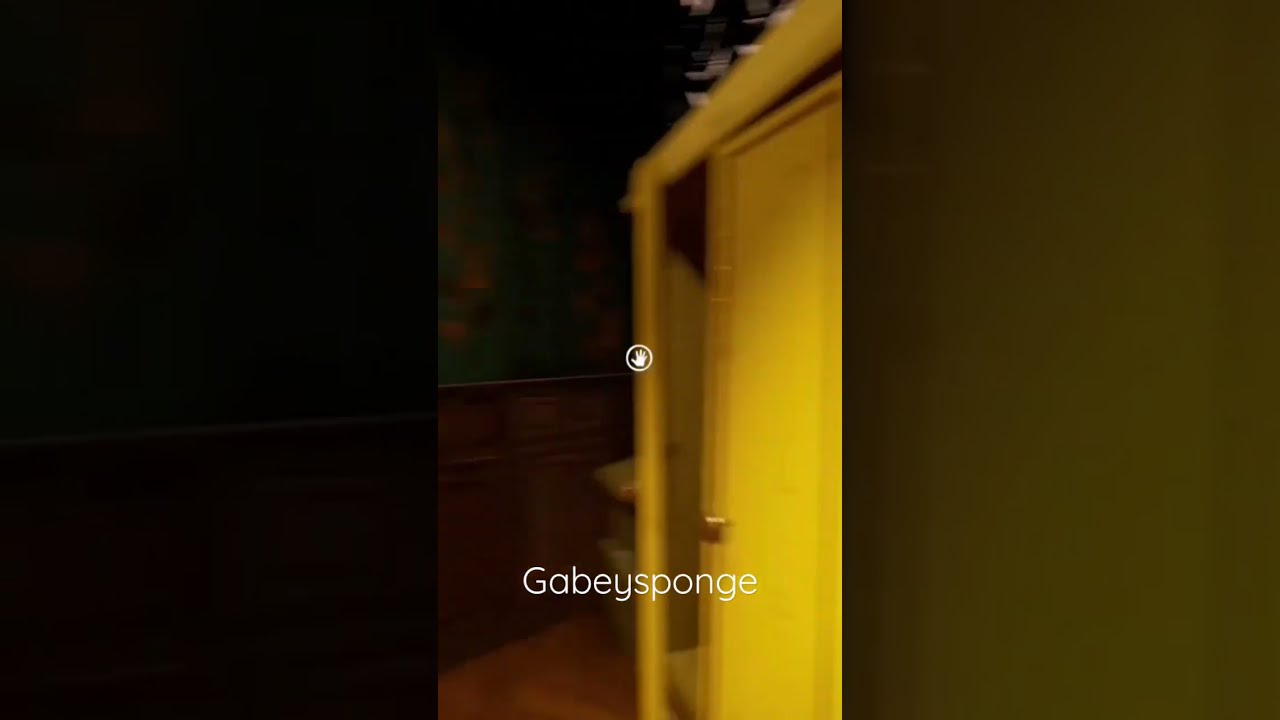The image is divided into three distinct vertical sections. The left third is completely black, representing a dark shadowed area, possibly the exterior of a building at night. The middle third contains a very blurry image of the inside of a home. This section features a poorly lit room with a half-open white door, which has a gold-colored handle and dark trim around its edges. The room has additional elements such as a brown cabinet, brown flooring, and a mixture of green and brown colors on the wall behind it. In the center of this blurry middle section is a small white circle containing a handprint. Near the bottom of this central area is white text reading "Gabby's Sponge." The right third of the image is a brownish-yellow rectangle, which appears to be a zoomed-in and faded continuation of the central section. The image is captured in a vertical cell phone style, emphasizing the indoor setting and the unclear, shadowy environment.